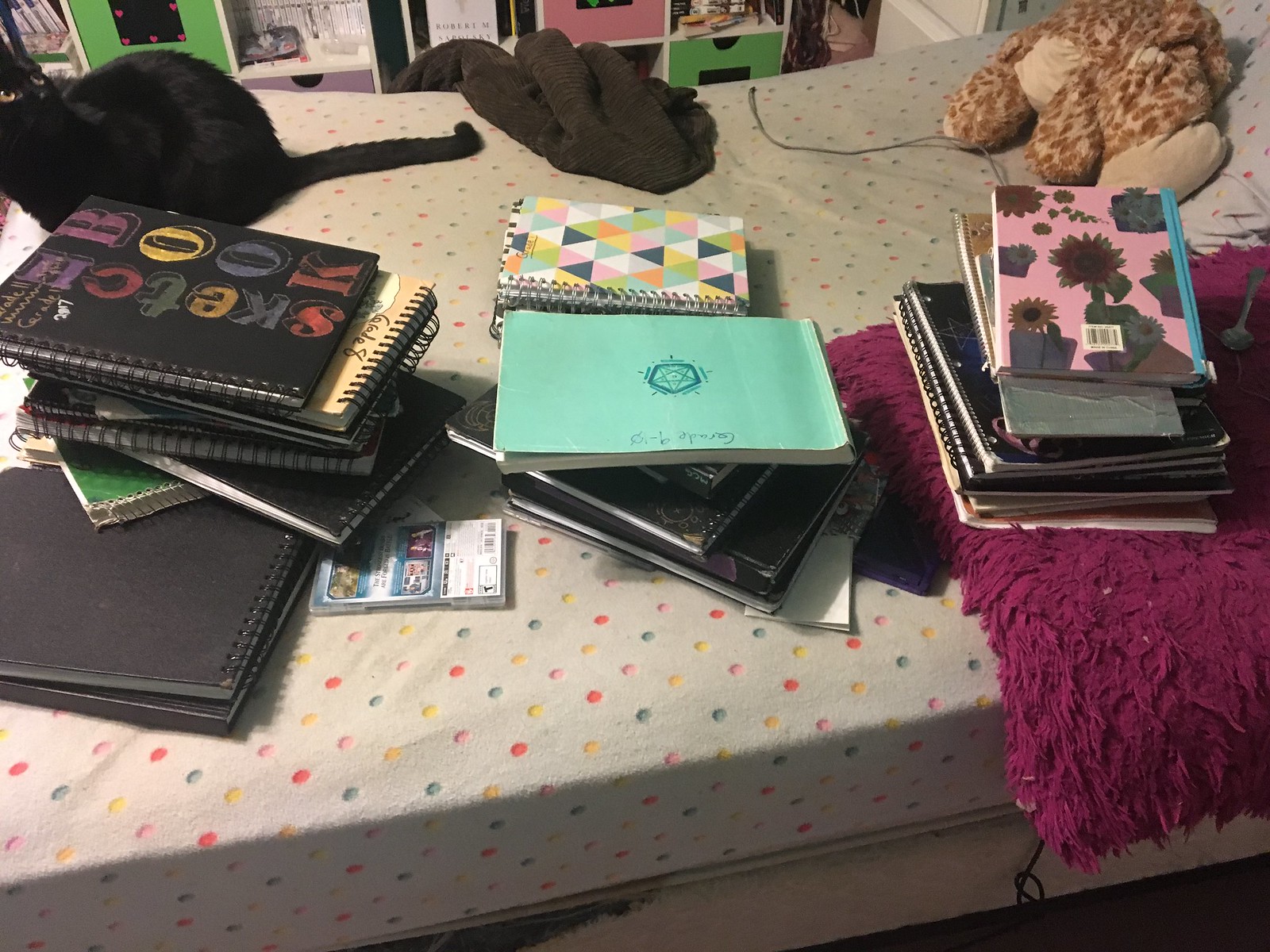The photograph depicts a twin bed adorned with a white sheet covered in multi-colored polka dots, encompassing hues of pink, blue, green, orange, and yellow. Scattered across the bed are four distinct stacks of sketchbooks, notebooks, and journals, some with spiral bindings and vibrant covers. Among them, the central stack features an assortment of binders and spiral-bound sketchbooks, including one identifiable by its checkerboard pattern. To the far left of the bed, another stack of spiral-bound books is topped by one with the word "Sketchbook" written in multi-colored letters. The rightmost stack holds a thin, hard-bound journal with a pink, floral cover resting on a piece of purple fabric that resembles shaggy, fake fur. An eclectic mix of additional items includes a stuffed giraffe placed at the head of the bed, a black jacket or sweatshirt draped midway across the bed, and a stack of books and notebooks positioned centrally. Completing the scene, a real black cat gazes upwards in the top left corner of the bed, adding a lively touch to the assortment. Shelves in the background further enhance the setting's cozy, lived-in ambiance.